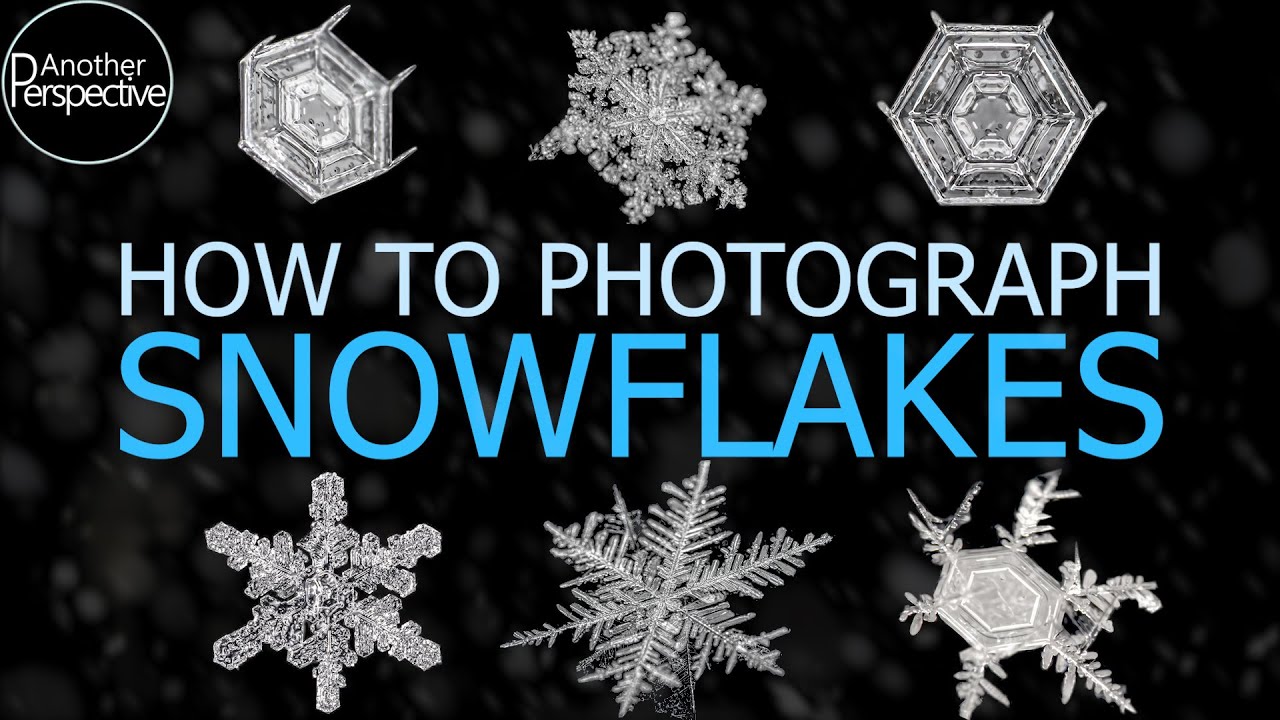The image appears to be a promotional banner for a course titled "How to Photograph Snowflakes." The design features a sleek black background dotted with blurry white spots, simulating a gentle snowfall. Dominating the center of the image is the large, two-tone green title text. In the top left corner, within a white circular watermark, is the name "Another Perspective," likely the organization or company promoting this course.

Prominently featured are six crystal-clear snowflakes, perfectly lit and sharply focused, showcasing their intricate and unique designs. The snowflakes are arranged with three at the top and three at the bottom. Those at the top exhibit a more solid, less branched structure, resembling square or diamond shapes. In contrast, the snowflakes at the bottom are more traditional, with long arms extending outward and detailed branching patterns. The overall impression is a meticulously crafted visual guide aimed at teaching the art of snowflake photography.